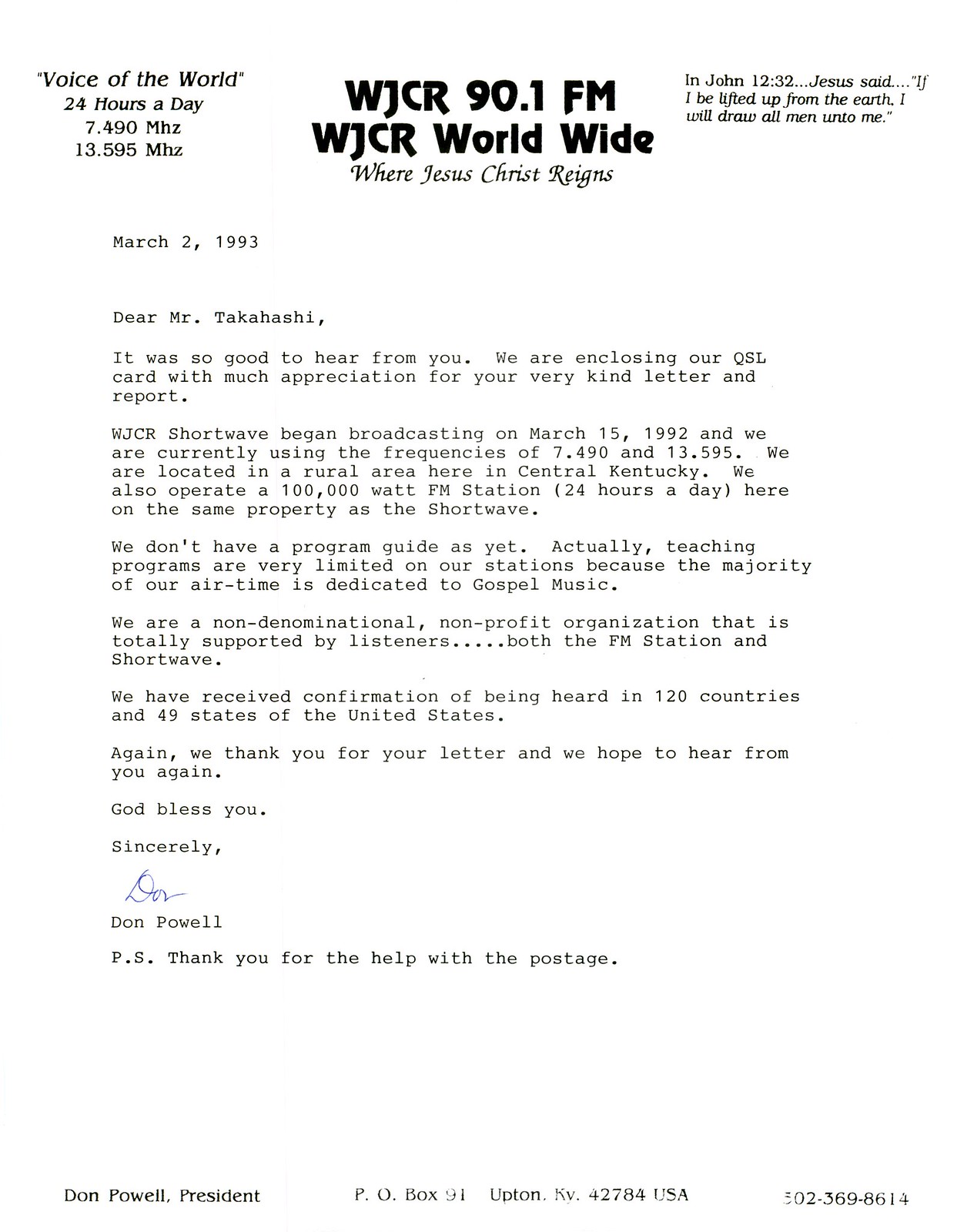The image is a portrait-oriented, black-and-white typed letter dated March 2, 1993. Positioned at the top in bold black lettering is "Voice of the World," indicating 24-hour broadcast frequencies at 7.490 MHz and 13.575 MHz. Adjacent to this on the left side is the logo "WJCR 90.1 FM, WJCR Worldwide," with a tagline beneath it stating, "Where Jesus Christ Reigns." On the right side, there is a biblical quote from John 12:32, "If I be lifted up from the earth, I will draw all men unto me."

Addressed to Mr. Takahashi, the letter acknowledges his kind correspondence and report, expressing gratitude and enclosing a QSL card. It mentions that WJCR began broadcasting on March 5, 1992, using the specified frequencies and running a 100,000-watt FM station alongside shortwave broadcasts from their rural central Kentucky location. The letter highlights that most airtime is dedicated to gospel music, with limited teaching programs, and notes that WJCR operates as a listener-supported, non-denominational, non-profit organization. The station has been received in 120 countries and 49 states. The letter concludes with gratitude, a blessing, and is signed in blue ink by Don Powell, who also thanks Mr. Takahashi for his assistance with postage. Address information appears at the end of the letter.